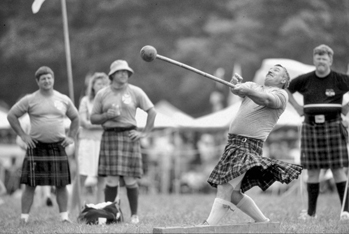This black and white photograph captures a lively scene at the Highland Games, a traditional Scottish sport event. In the foreground, four men are standing on a grassy field, all dressed in short-sleeved T-shirts and plaid kilts. The central figure is intensely focused, swinging a heavy ball attached to a long stick or chain, preparing for an imminent throw. His kilt flutters in the wind, revealing tight white boxer shorts and tall, white knee-high socks. Flanking him to the right is another man observing the action, while two more men with hands on their hips stand to the left. Nestled between them is a woman wearing a white skirt. In the background, partially obscured and out of focus, are tents and canopies, hinting at the festive atmosphere of the event, with faint outlines of hills or woodland beyond.